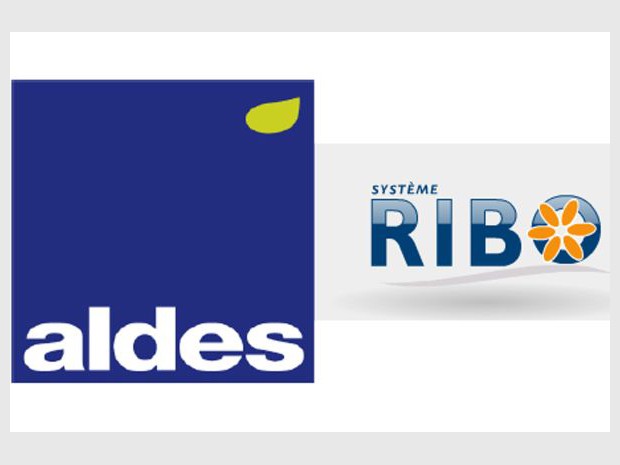The image features two distinct logos centered within a white rectangle, bordered by a light gray frame that's thicker on the top and bottom and thinner on the sides. On the left side of the rectangle is a solid blue square logo, adorned with a green, leaf-shaped icon in the upper-right corner. Beneath the leaf, the text "ALDES" (spelled A-L-D-E-S) is displayed in white. To the right of this blue logo is a gray rectangular logo featuring a gradient that transitions from dark gray at the bottom to light gray at the top. In this rectangle, the word "SYSTÈME" is written in smaller blue text with an accent mark over the last 'E.' Below "SYSTÈME," the larger word "RIBO" is also in blue, fading to white at the top. At the top of the 'O' in "RIBO," there is a star pattern made of six orange ovals, resembling a flower. The overall arrangement appears to be graphical, possibly resembling a presentation slide or advertisement, featuring colors such as gray, white, blue, orange, and green.